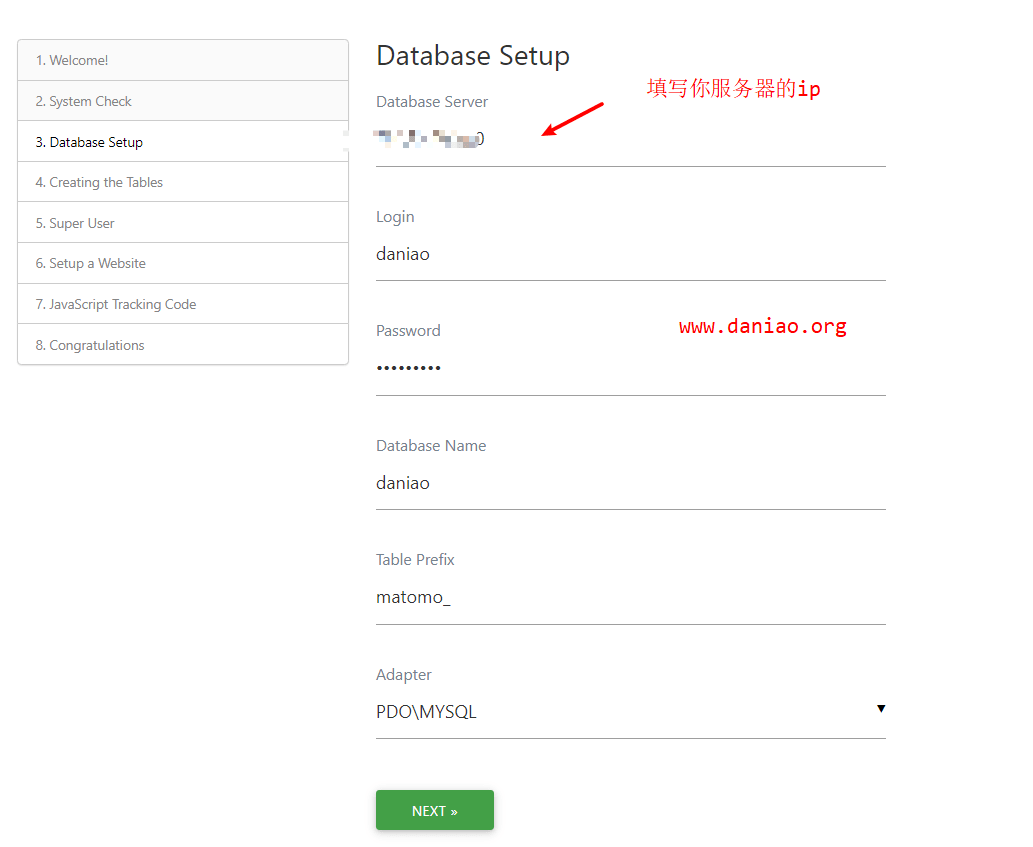A detailed screenshot of a website's desktop interface, seemingly formatted partially like a mobile site. The current screen is part of a database setup section, as indicated by the header "Database Setup" prominently displayed. The interface features a left pane with a series of selectable options, arranged sequentially to guide the user through the setup process, resembling a structured wizard or guide. There are a total of eight steps outlined: Welcome, System Check, Database Setup, Creating the Tables, Super User, and other subsequent steps necessary for a complete setup.

Currently highlighted is step three, "Database Setup," which requires the user to fill in multiple fields with technical information: Database Server, Login, Password, Database Name, and Table Prefix. Each field is essential for configuring a functional database, indicating a formal and structured setup approach typical of database management systems. Additionally, there's a section of red text displayed on the screen, written in Japanese characters, whose purpose is unclear but may imply an error message or important instruction in a foreign language. This intricate setup screen is indicative of the technical and precise nature of establishing a back-end database configuration.